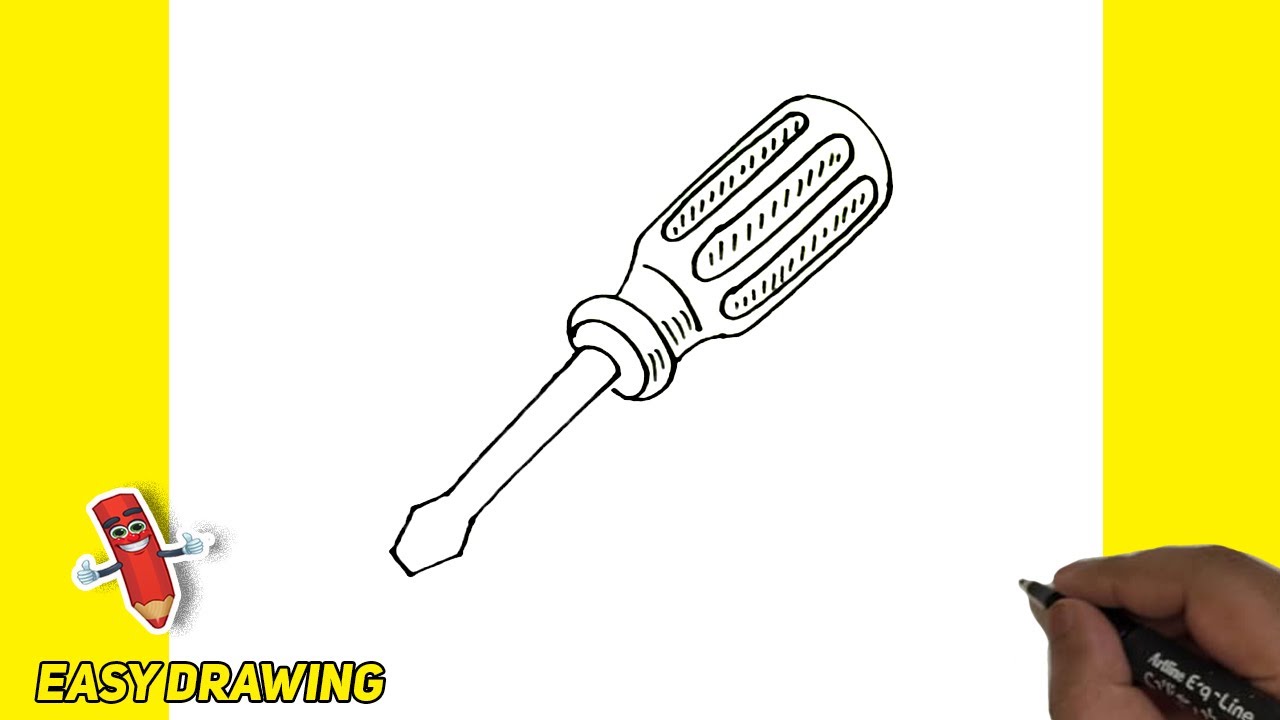The illustration appears to be a YouTube thumbnail titled "Easy Drawing," showcased in yellow bubble letters at the bottom left corner. A cheerful animated red pencil with white teeth, black eyebrows, black and white eyes, and small white-gloved hands giving a thumbs up is positioned above the text. The central focus of the image is a hand-drawn black and white line art of a screwdriver, outlined with thick ink. This drawing is realized on what looks like a piece of paper, highlighting its hand-crafted essence. In the bottom right corner, a dark hand holding a pen or pencil contributes to the hand-drawn theme. The composition is framed by yellow stripes or borders on the left and right sides, adding a balanced structure to the overall layout.